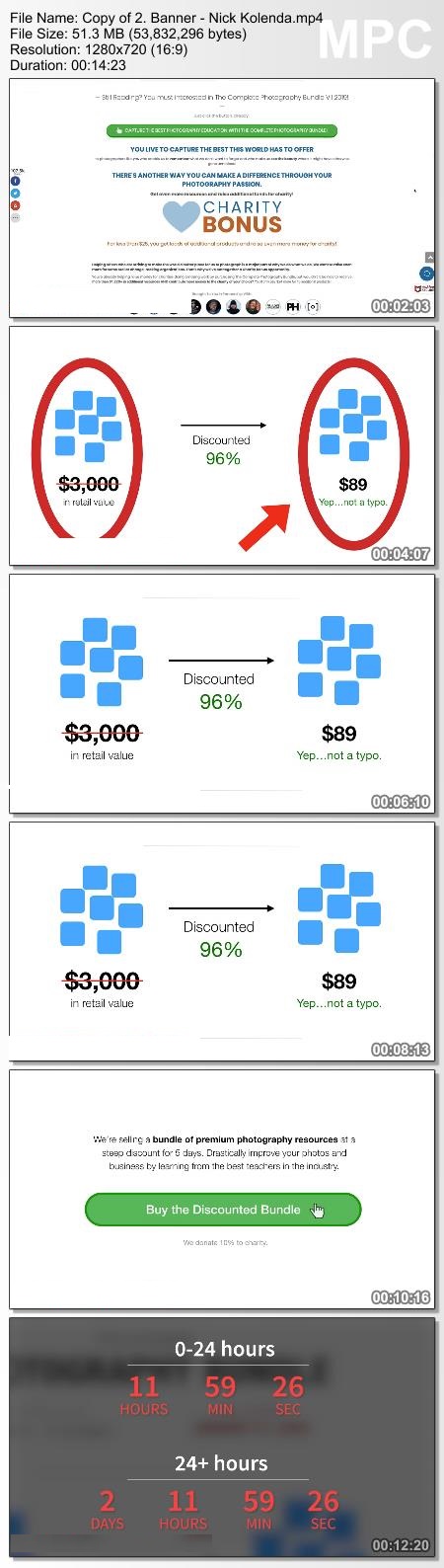The image depicts an advertisement for a charity-driven promotion aimed at photography enthusiasts. It prominently features a bold headline, "Charity Bonus," emphasizing the philanthropic nature of the offer. The text introduces the opportunity for individuals to make a positive impact through their passion for photography. 

A $3,000 retail value is strikingly crossed out with a red line, and a big arrow in red points to the new discounted price of just $89, highlighting the incredible deal. The advertisement clarifies that the discount is indeed not a typo and represents a significant savings of over 96%.

Additionally, the bottom right corner of the image includes sequential timestamps such as "00:04:07," "00:06:10," and "00:08:13," possibly referencing specific sections or products within bundled offers.

Finally, the caption at the bottom promotes a limited-time offer, valid for five days only, to purchase a bundle of premium photography resources. This bundle promises to drastically improve both photography skills and business acumen, with guidance from top industry professionals. The message is reinforced with urgency, noting the time left, "10:16:02" and "24 hours 11 minutes 59 seconds," indicating the countdown to the end of the promotion.

Overall, the caption emphasizes the value, urgency, and charitable aspect of the offer, enticing photography enthusiasts to act quickly to secure the deeply discounted resources.